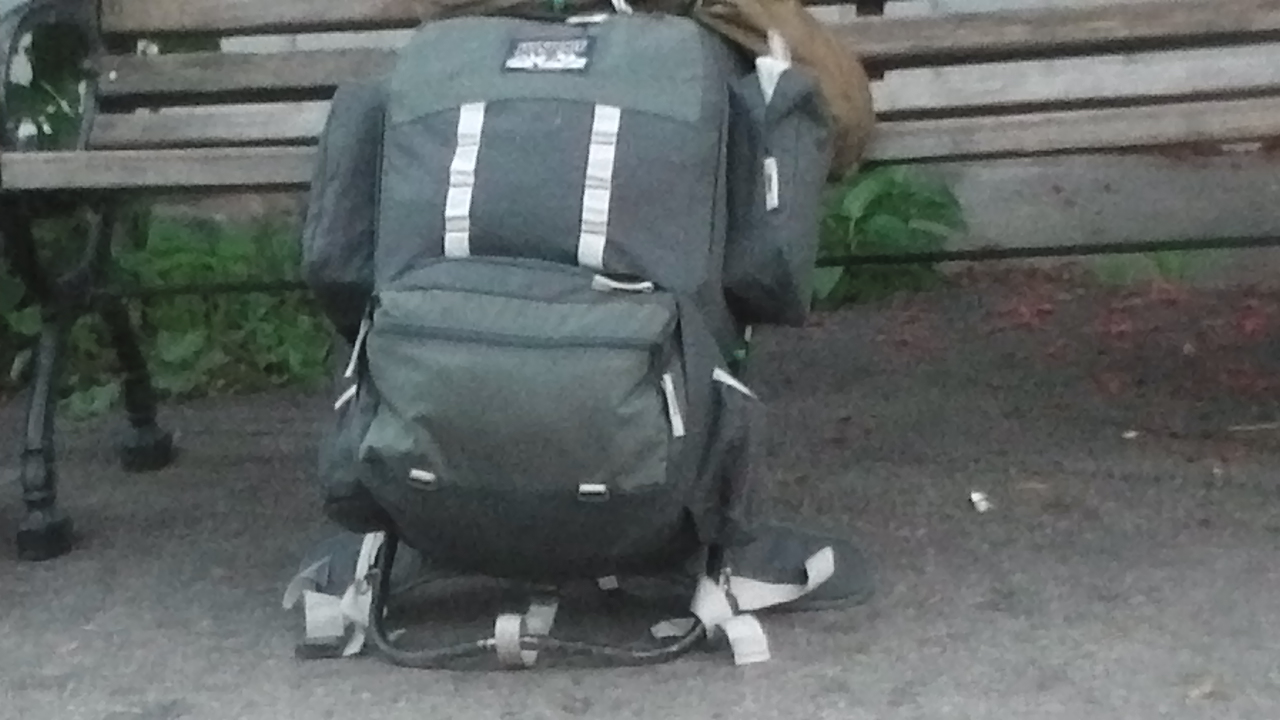This is a color photograph taken outdoors in a park. It showcases a large, hikers' backpack leaning against a weathered park bench. The backpack is primarily a muted green with whitish silver stripes and darker green areas, indicative of heavy use and exposure to the elements. It features one small front pouch, a large central compartment, and two side pockets, providing ample storage space suitable for a weekend camping trip. Detailed with white and light gray straps, the backpack is supported by a slightly worn metal frame designed to prevent tipping.

The park bench, constructed from a light, weathered wood, rests on a dark blackish-gray concrete or tarred surface. The bench’s base is held up by X-shaped black metal legs with connecting rods running underneath. Surrounding the bench and backpack are green plants and dark brown leaves scattered on the ground, suggesting a fall season. The scene conveys a tranquil, rustic environment with no people present, allowing focus on the well-prepared backpack amidst the natural park setting.